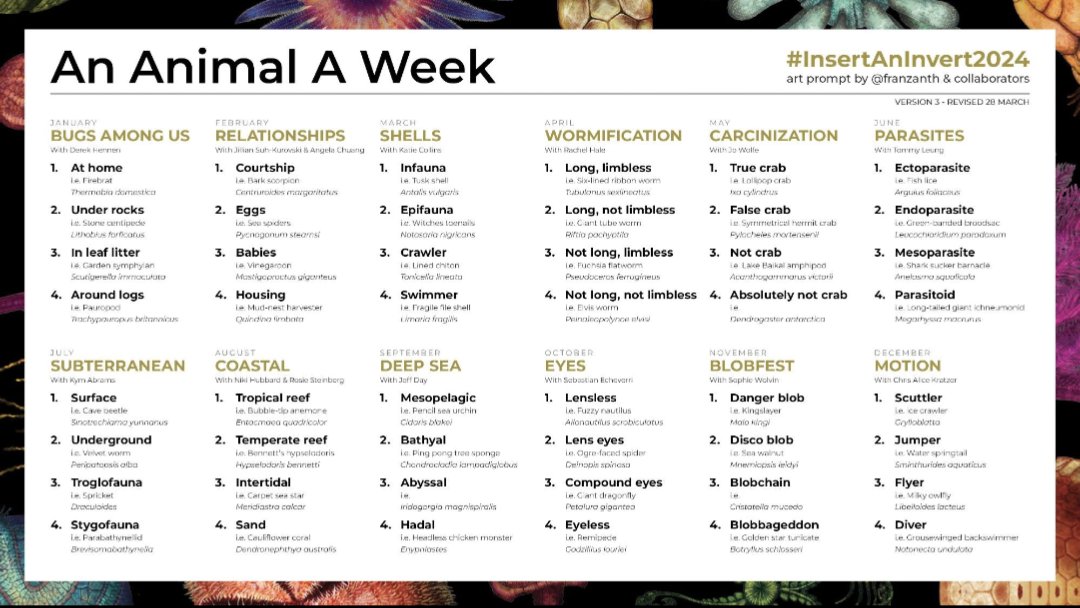This detailed, colorful infographic titled "An Animal a Week" serves as the 2024 art prompt by @FranzAnth and collaborators. The chart is version 3, revised 28 March, and features a white sheet of text overlaying a flowery background. At the top right, it includes the hashtag #InsertandInvert2024. Each month from January to December is assigned a specific theme related to the animal kingdom, with four weekly prompts underneath each heading.

- **January: Bugs Among Us** – Topics include at home, under rocks, in leaf litter, around logs.
- **February: Relationships** – Focuses on courtship, eggs, babies, housing.
- **March: Shells** – Includes infauna, epifauna, crawlers, and swimmers.
- **April: Warmification** – Features variations of limbless and long, not limbless, not long combinations.
- **May: Carcinization** – Explores true crabs, false crabs, not crabs, and absolutely not crabs.
- **June: Parasites** – Covers ectoparasites, endoparasites, mesoparasites, and parasitoids.
- **July: Subterranean** – Looks into surface, underground, troglofauna, and stigofauna habitats.
- **August: Coastal** – Delves into tropical reef, temperate reef, intertidal, and sand environments.
- **September: Deep-Sea** – Examines mesopelagic, bathyal, abyssal, and hadal zones.
- **October: Eyes** – Describes lensless, lens eyes, compound eyes, and eyeless species.
- **November: Blobfest** – Introduces danger blob, disco blob, blob chain, and blobageddon.
- **December: Motion** – Encompasses scuttlers, jumpers, flyers, and divers.

For each theme, additional topics are provided for each of the four weeks, making it a thorough and engaging art prompt schedule that runs throughout the year.